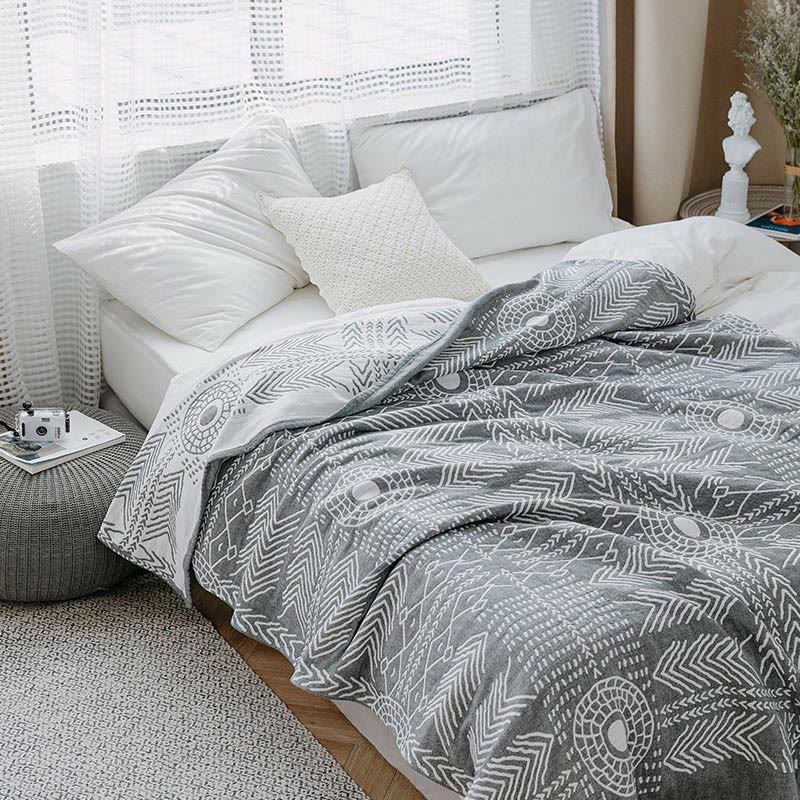This square-shaped photograph captures a professionally taken image of a bedroom, with a bed as the central focus. The bed appears to be queen-sized, adorned with an intricate patterned gray comforter featuring white stripes, lines, dots, circles, and unique shapes resembling chicken scratch marks. The comforter is two-sided with one side having a dark gray background and light gray pattern and the other side having a white background with dark gray pattern. Three pillows – two large white ones and one smaller pillow in between – are unneatly placed at the top of the bed, indicating it was recently used.

Over the bed, a white curtain partially covers two windows, allowing a hint of light to seep through. To the left of the bed sits a small gray ottoman or cushion with a DSLR camera and a book or magazine placed on top. On the right side, a marble Masonic statue and a plant are situated on a nightstand, with another magazine underneath the plant. A gray rug lies below the bed, anchoring the serene and slightly disordered ambiance of the room.